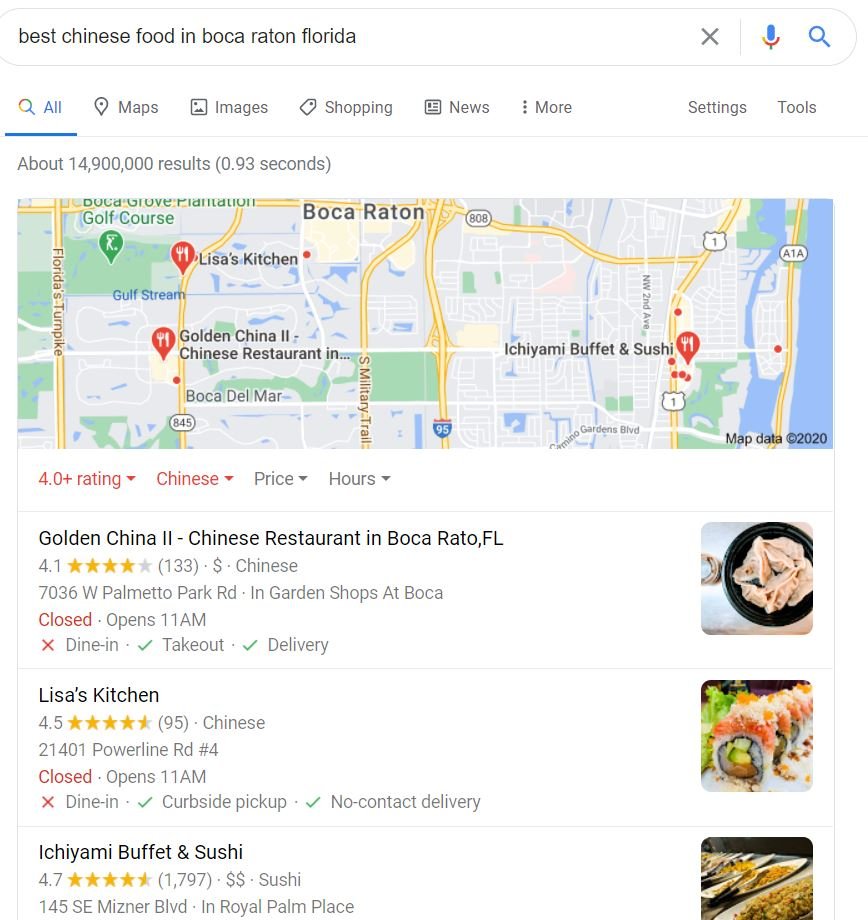**Caption:**

The image depicts a screenshot from a search engine highlighting the search query "best Chinese food in Boca Raton, Florida." At the top of the page, the search bar displays the typed query in black text, accompanied by an "X" symbol, a microphone icon, and a magnifying glass icon for search. Below the search bar, a navigation menu includes underlined "All" followed by "Maps," "Images," "Shopping," and "News," with "More" displayed next to three vertical dots.

The search results indicate approximately 14,900,000 findings in 0.93 seconds. A map of Boca Raton is shown, pinpointing various Chinese restaurants in red markers, while other landmarks are tagged in green. Waterways and geographical details are also visible.

Beneath the map, a filter text specifies "4.0+ rating, Chinese, price, hours." The top result lists "Golden China," a Chinese restaurant rated 4.1 stars. Details reveal it is currently closed, with an opening time of 11 a.m., and offers dine-in, takeout, and delivery services.

Next is "Lisa's Kitchen," boasting a 4.5-star rating from 995 reviews. The restaurant specializes in Chinese cuisine, provides the address, and highlights options for dine-in, curbside pickup, and no-contact delivery. It is also currently closed and opens at 11 a.m.

The third listing features "Ichiyami Buffet and Sushi," noted as "I-C-H-I-Y-A-M-I" and rated 4.7 stars from 1,797 reviews. It is categorized under sushi and includes the address details.